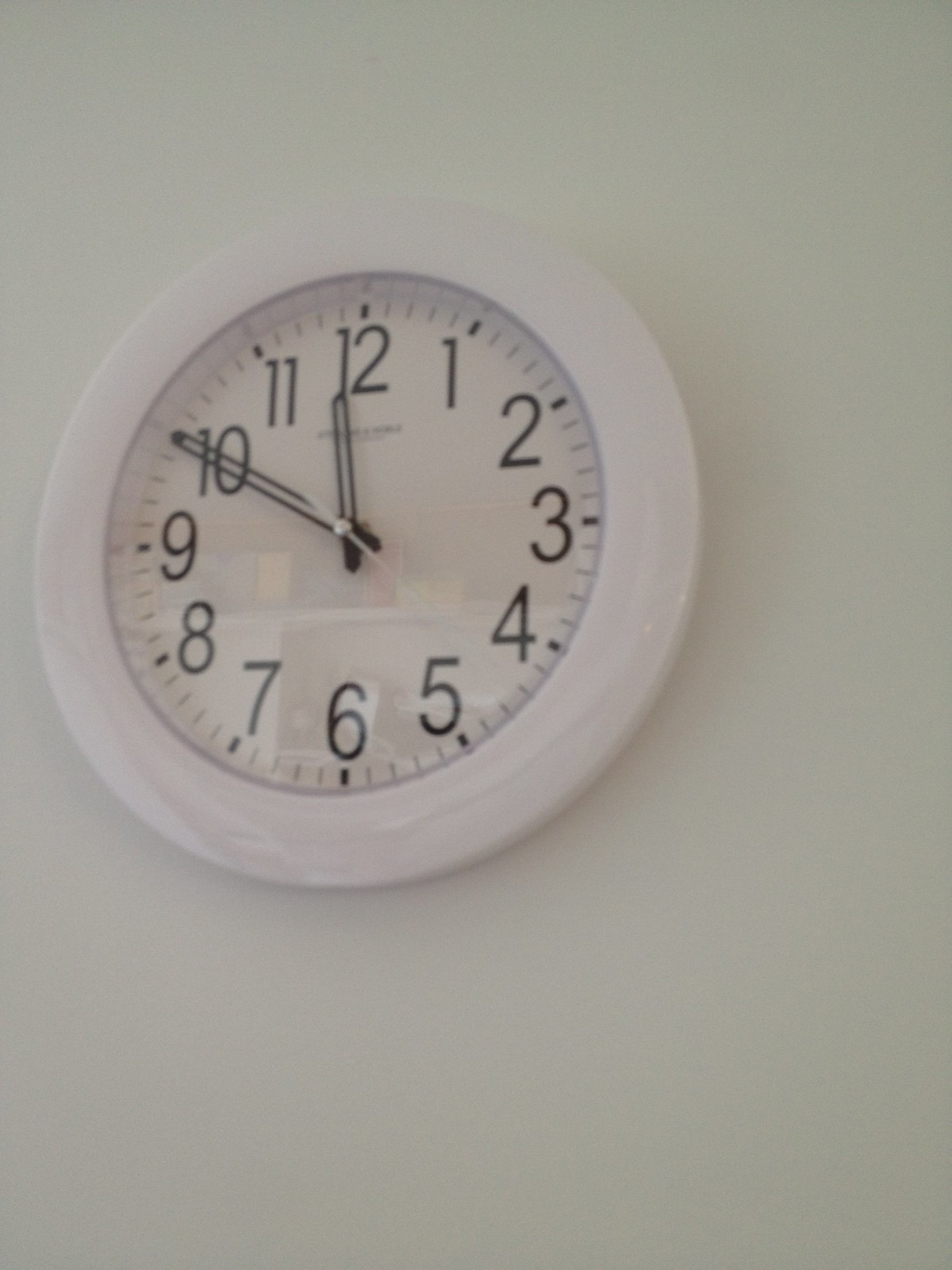This color photograph captures a round, white clock prominently displayed slightly to the left of center. The clock, which takes up about half the width and height of the image, has a glossy, thick white border that could be made of either plastic or metal. Just inside the border, a faint gray design is visible. The clock face features black numerals in the standard numerical format from 1 to 12, and minute markers are indicated by small lines between the numbers.

The hands of the clock are distinct and black, with the hour hand being shorter and the minute hand approximately two-and-a-half times longer. Both hands are hollowed out rather than solid. The second hand is incredibly thin and white. The time displayed is around 11:50, or 10 minutes to 12. 

There is a vague reflection on the clock's surface showing hints of yellow and pink, though the source of the reflection is indiscernible. The wall behind the clock is a muted, whitish-green, and a shadow is cast to the right of the clock, suggesting the light source is coming from the left. The overall palette is subdued, making the image appear almost like an illustration rather than a photograph. Additionally, the clock might have the manufacturer's name, but it is too small and out of focus to read.